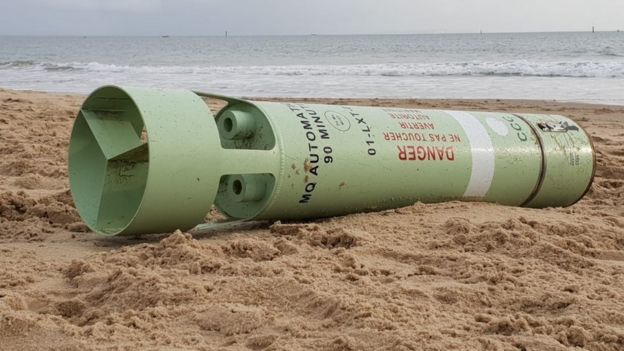In this detailed image, we observe a French warning label on what appears to be a bomb or bomb disposal device, strategically placed on a beach. The device, resembling a torpedo, is a long, slender steel tube, evocative of an unusually elongated fire extinguisher. It is painted a pale green color. Toward the rear end, the tube transitions into a propeller-like structure supported by struts, giving it a unique and somewhat ominous appearance.

Prominently displayed on the side of the device is the word "DANGER," accompanied by the French warning "Ne pas toucher" (do not touch). Although more text is present, it becomes increasingly difficult to read. These warnings indicate the potential for the device to explode if tampered with.

A white line is marked across the lower section of the device. Nearby, an observable segment appears designed to be unscrewed, a feature likely intended for placing or removing an explosive payload. This implies that the device may house explosive materials within, meticulously sealed to ensure that, if detonated, the explosion’s force and shrapnel are channeled through three small segmented holes and the fan-shaped exit, potentially serving to minimize the impact.

The presence of such a device, particularly on a public beach, emphasizes the gravity of the warning labels and the necessity to heed such cautions diligently to avoid catastrophic consequences.